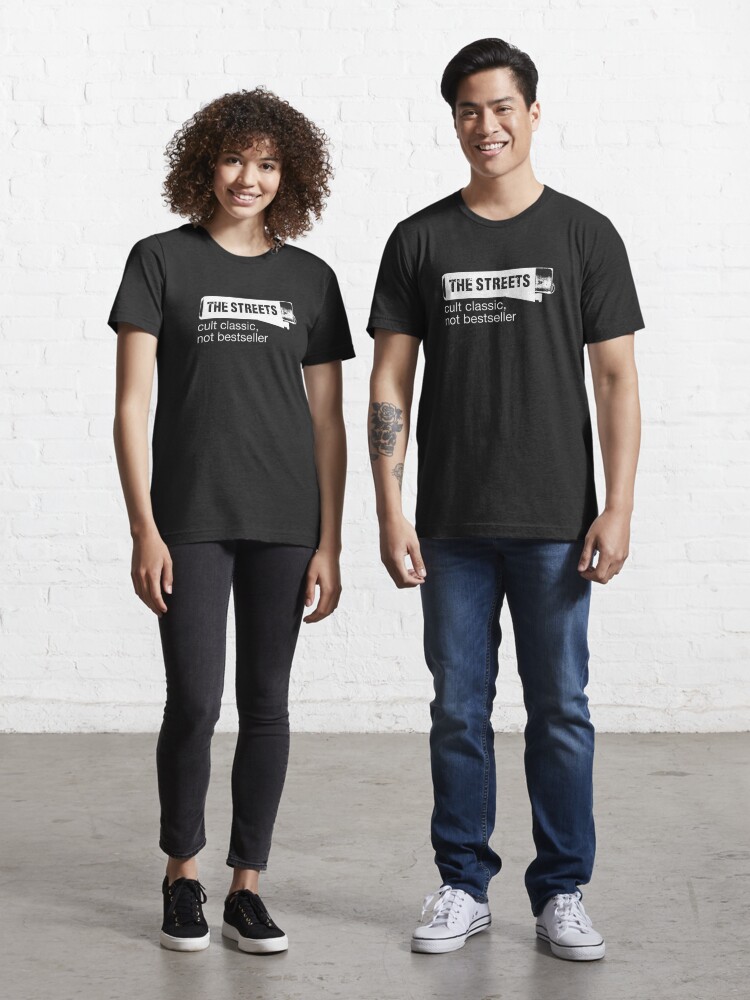This indoor photographic image captures a young Asian man and a young woman, likely of mixed Black and White heritage, standing next to each other against a white-painted brick wall. The wall spans approximately three-fourths of the image, with a light gray, concrete floor occupying the lower fourth of the picture. 

The man on the right is smiling warmly at the camera, showcasing his short, neatly trimmed, slicked-back hair parted on the left side. He is dressed casually in a black t-shirt that reads "The Streets" in dark text within a white rectangle, followed by "cult classic, not bestseller" beneath it, paired with blue jeans and white sneakers, resembling Chuck Taylors. A distinctive tattoo of a skull entwined with a rose adorns his right forearm just below the elbow.

Standing to his left is the woman, also smiling at the camera, her curly, light brown hair framing her face and descending to her neck. She mirrors his casual style with an identical black t-shirt emblazoned with "The Streets" and the same slogan. She completes her outfit with form-fitting black pants, resembling slim or black leggings, and black sneakers, likely Vans, noticeable for the absence of visible socks. Their casual stances, with arms hanging by their sides, against the stark, industrial background, evoke a relaxed, urban vibe.